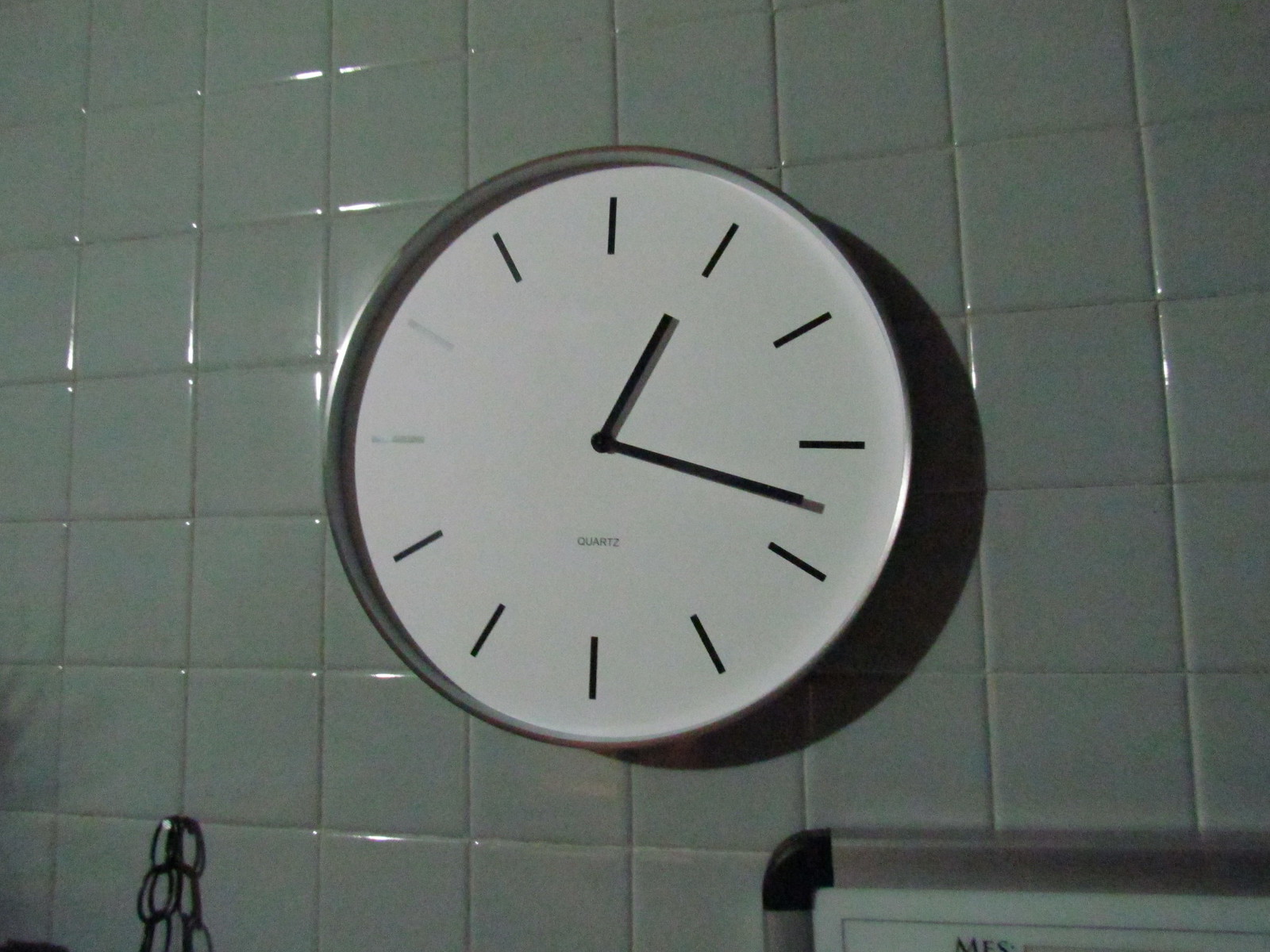This photograph depicts a wall-mounted analog clock with a minimalist design. The clock features a metal, likely silver, housing and a pristine white face devoid of numerals, marked instead by simple black dashes to indicate the hours. Notably, the dashes at the 9 and 10 positions appear silver, likely due to reflective light. The clock's hour and minute hands are basic black rectangles, with the minute hand pointing between the 3 and 4, and the hour hand on the 1, indicating the time is either 1:20 or 12:20. The word "QUARTZ" is printed in small, uppercase letters just above the 6. 

The clock is set against a background of small, greenish-teal square tiles with light gray grout, adding a distinctive texture to the setting. A silver chain hangs from the bottom left corner, attached to the wall. Additionally, part of a framed item with black and silver elements is visible on the right side of the image. The scene is illuminated by light reflecting off both the clock’s face and the tiles, suggesting a well-lit environment.